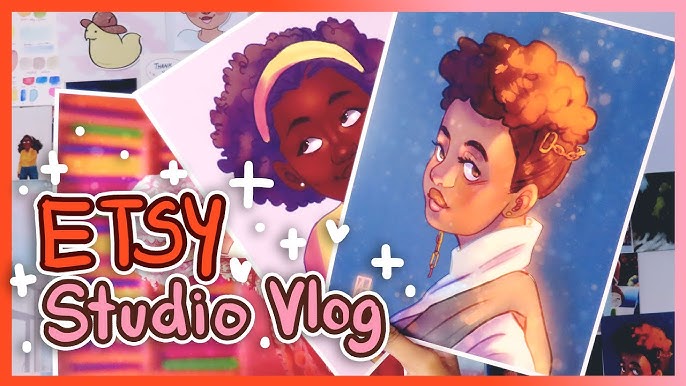This image appears to be an advertisement featuring a vibrant and artistic design. The focal point is the text that reads "Etsy" in bold, bobbly font with a black outline and a white border, and "Studio Vlog" below it in pink. The background gradient transitions from red to pink on one side.

The centerpiece of the ad consists of two overlapping illustrations of African-American women, depicted in a cartoon style. The front illustration, against a blue backdrop, shows a woman with lighter skin, curly hair, a brown vest, and a white undershirt, looking directly at the camera from a side angle. The second illustration, partially obscured and set against a white background, reveals a woman with darker skin, a yellow headband, and puffy hair, gazing upwards with a sly smile.

Additional elements scattered in the background include various artistic pieces, such as a small image resembling a duck with a hat and miniatures of the women in the primary illustrations. The entire composition is framed with a pink and orange border, and the overall layout evokes a creative, hand-drawn aesthetic, making it a striking advert for Etsy Studio Vlog.